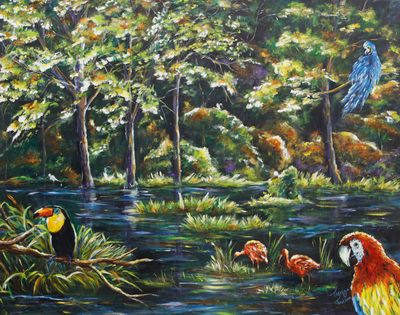This vibrant, full-color painting depicts a lush, jungle-like landscape with a dark blue marsh or stream running through the bottom to the middle of the square canvas. The scene, bathed in daylight with sunlight filtering through the leaves, showcases an array of exotic birds and verdant flora. In the lower right-hand corner, a striking red, blue, and yellow parrot with a white face perches prominently. Just to its left, a pair of elegant flamingos wade in the water amid small plants. To the far left, another exotic bird—a black-bodied toucan with a yellow head, blue eyes, and an orange beak—adds to the tropical diversity. An additional blue bird is situated in the upper right corner, perched on a branch. Tall trees with brown trunks rise in the background, adorned with leaves in shades of green, white, and orange, interspersed with thick shrubbery and low-lying grasses emerging from the water. The painting seamlessly merges its elements to create a stunning representation of a vibrant natural habitat, though the artist remains unidentified.